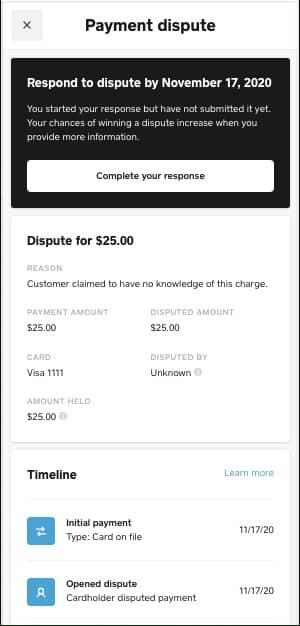This screenshot captures the detailed contents of a payment dispute pop-up box from a credit card company website. In the upper left corner, there is a gray box featuring an "X" icon for closing the pop-up. Centered at the top, the header reads "Payment Dispute" in bold black letters. Directly below the header, a black notification box alerts the user with the message, "Respond to dispute by November 17th, 2020."

Further down, in smaller white text within another black box, it states: "You started your response but have not submitted it yet. Your chances of winning a dispute increase when you provide more information." At the bottom of this section, within a white bar, there is a call-to-action button labeled "Complete your response."

Below this bar, details of the dispute are presented within another white box. It specifies that the dispute is for a $25 transaction, citing the reason as the customer claims to have no knowledge of the charge. The section lists the disputed amount ($25), the card type, and the last four digits of the card number. It notes that the dispute was filed by an "unknown" individual, with an amount of $25 being held.

At the very bottom of the pop-up, a titled section labeled "Timeline" provides a chronological summary on the right-hand side. At the top right corner of this section, a "Learn More" hyperlink is present. Below that, two entries are listed: 
1. Initial Payment: Type - Card on File, Date - 11/17/20.
2. Open Dispute: Card holder disputed payment, Date - 11/17/20.

These details provide a comprehensive overview of the dispute process and the current status of the queried transaction.